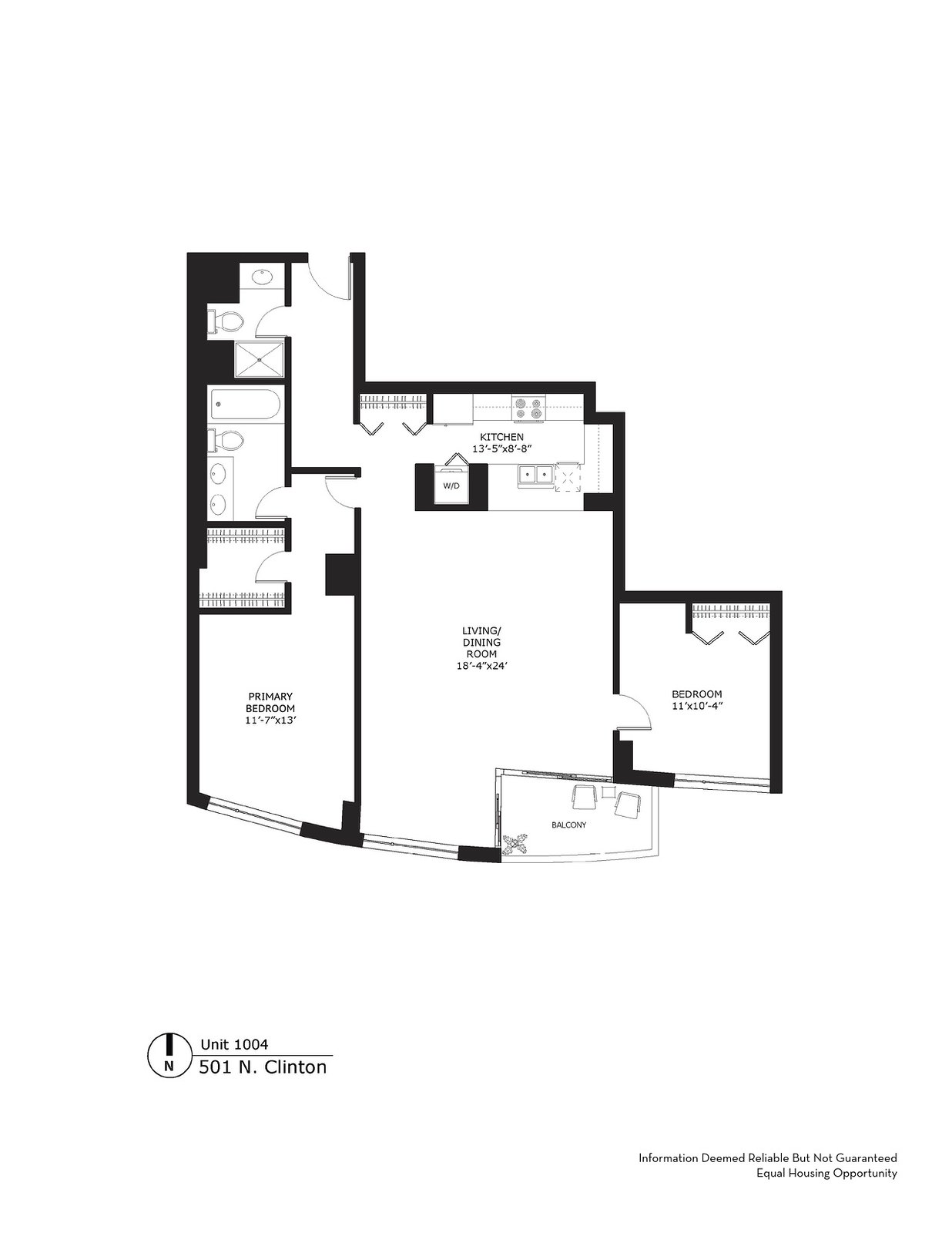This detailed caption describes a top-down, computer-designed floor plan for Unit 1004 at 501 North Clinton. The image is marked with a circle and an upward-pointing arrow indicating the north direction. In the bottom right corner, there is a disclaimer stating "Information deemed reliable but not guaranteed. Equal Housing Opportunity."

The layout features a front-facing balcony, which includes a small potted plant, two chairs, and a table between them. Directly behind the balcony is a spacious living/dining room area, measuring 18 feet 4 inches by 24 feet. To the right of the dining room is a door leading to a bedroom that measures 11 feet by 10 feet 4 inches. This bedroom is unfurnished but includes a south-facing window and a closet with accordion-style doors.

Adjacent to the rear of the living room is the kitchen, which measures 13 feet 5 inches by 8 feet 8 inches. The kitchen is equipped with a stove, a sink, possibly an additional appliance, and a pantry-like closet similar in design to the bedroom closet. From the kitchen, a door leads to an unspecified area beyond the plan's scope. Next to this door is a small, unlabeled bathroom containing a sink and a toilet.

Returning to the living/dining room, another door opens into the primary bedroom, which measures 11 feet 7 inches by 13 feet. This bedroom features a large closet and an adjoining master bathroom. The master bathroom, though unlabeled, includes a bathtub, a toilet, and two sinks.